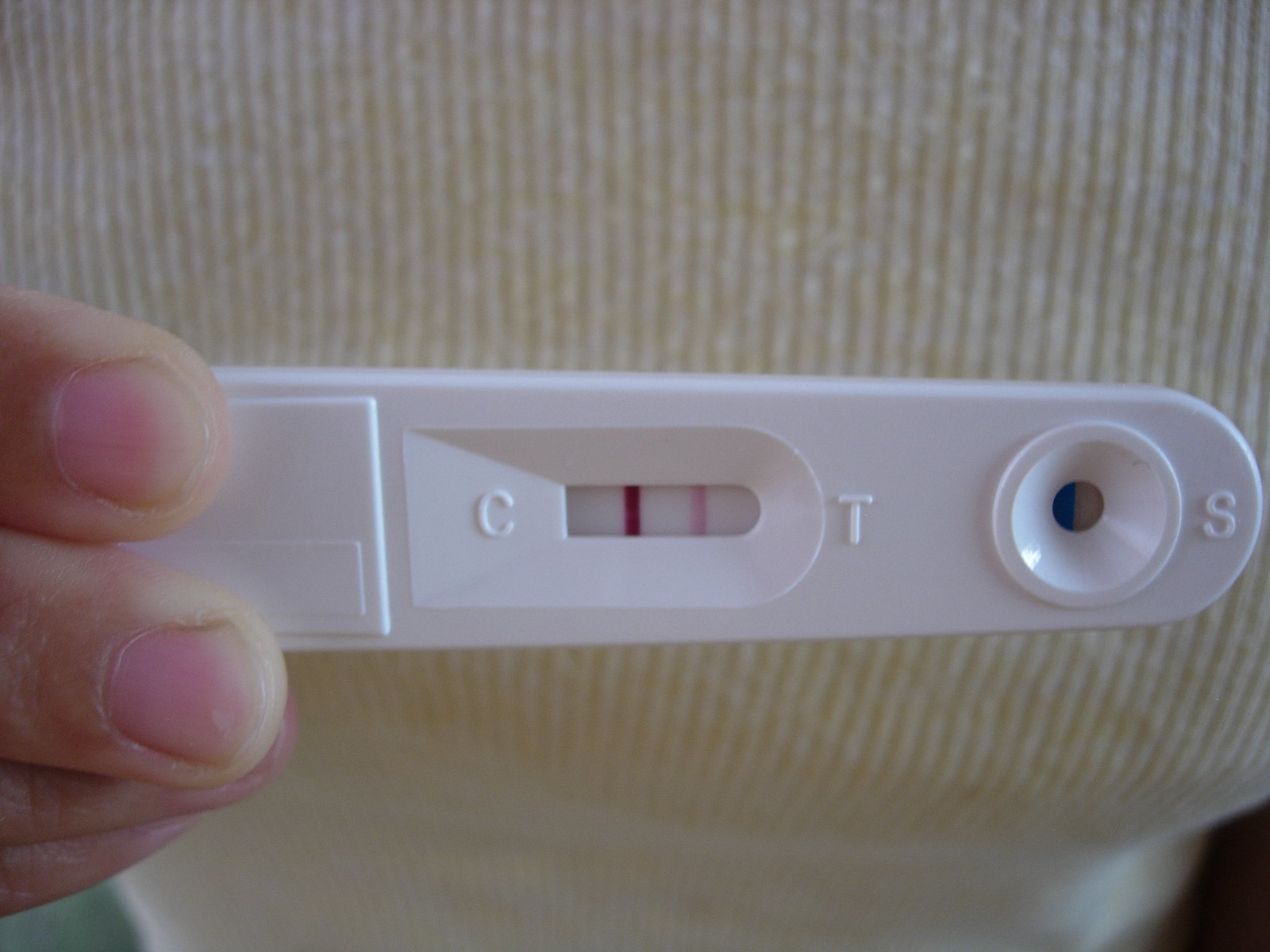In this color landscape photograph, a positive COVID-19 test prominently occupies the center of the frame. The white, smooth-edged, rectangular test device lies horizontally, displaying one distinct red line by the "C" and another by the "T," indicating a positive result. The test is being held by a woman's right hand, partially visible with her fingers gripping the device carefully. The background features the woman's chest, slightly busty, clothed in a cozy, yellow wool shirt. The focus of the image is unmistakably on the test, capturing a moment of revelation and reflection.